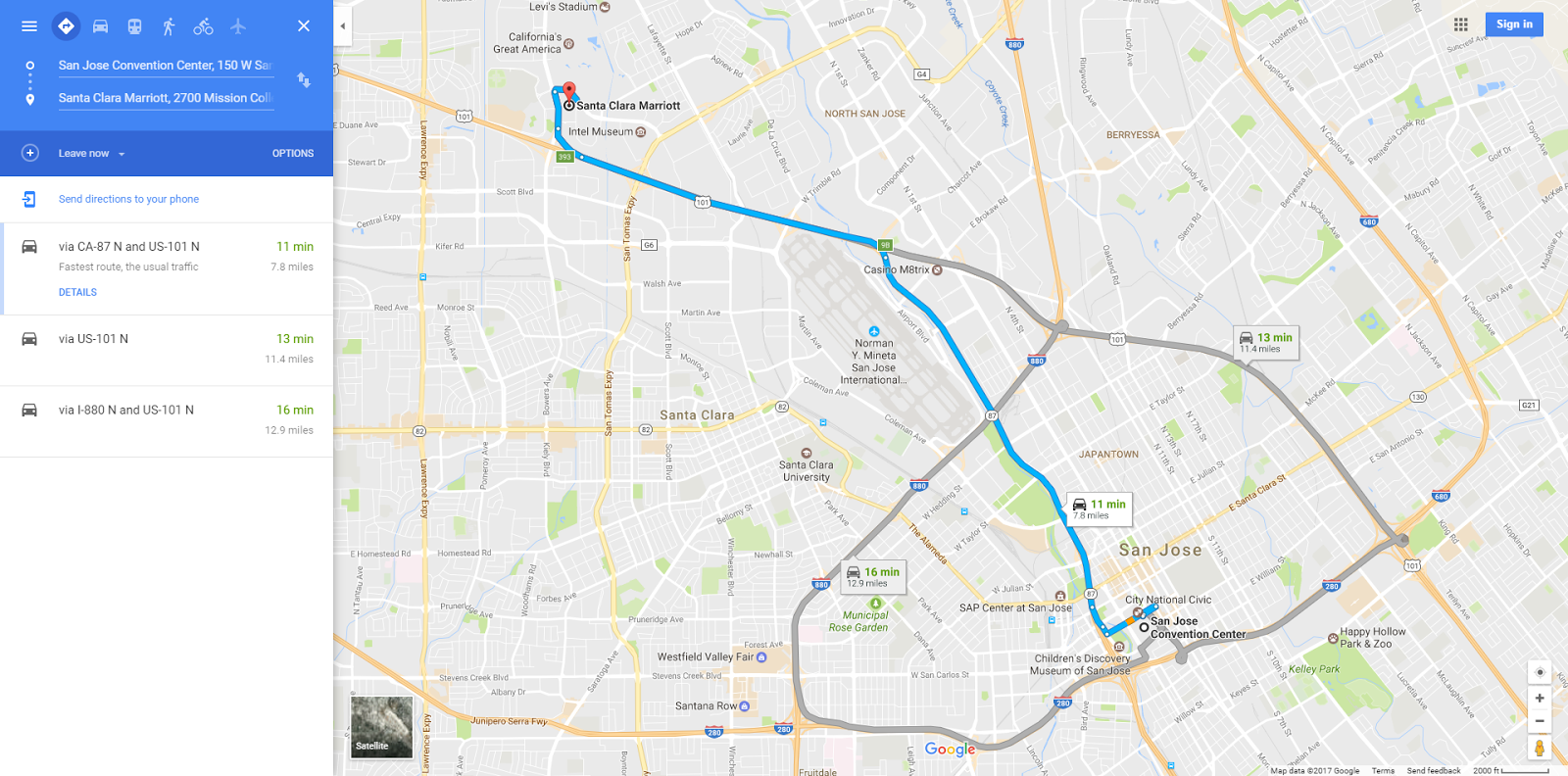This image shows a landscape-oriented screenshot of the Google Maps website, clearly detailing a navigation plan. To the left side of the screen, a vertical information box is displayed. This box includes the starting point, San Jose Convention Center, and the destination, Santa Clara Marriott. It outlines various travel options including driving, public transportation, walking, cycling, and air travel. Currently, the driving option is selected, set to depart immediately.

The box further lists three possible driving routes, indicating travel times of 11 minutes, 13 minutes, and 16 minutes respectively. The fastest route, highlighted in blue, is selected, while the other two routes are displayed in gray.

On the right side of the screen is a large, detailed map. It shows the geographical layout, street names, and the marked routes. The selected blue route stands out prominently against the less emphasized gray alternatives, providing a clear visual guide from the starting point to the destination.